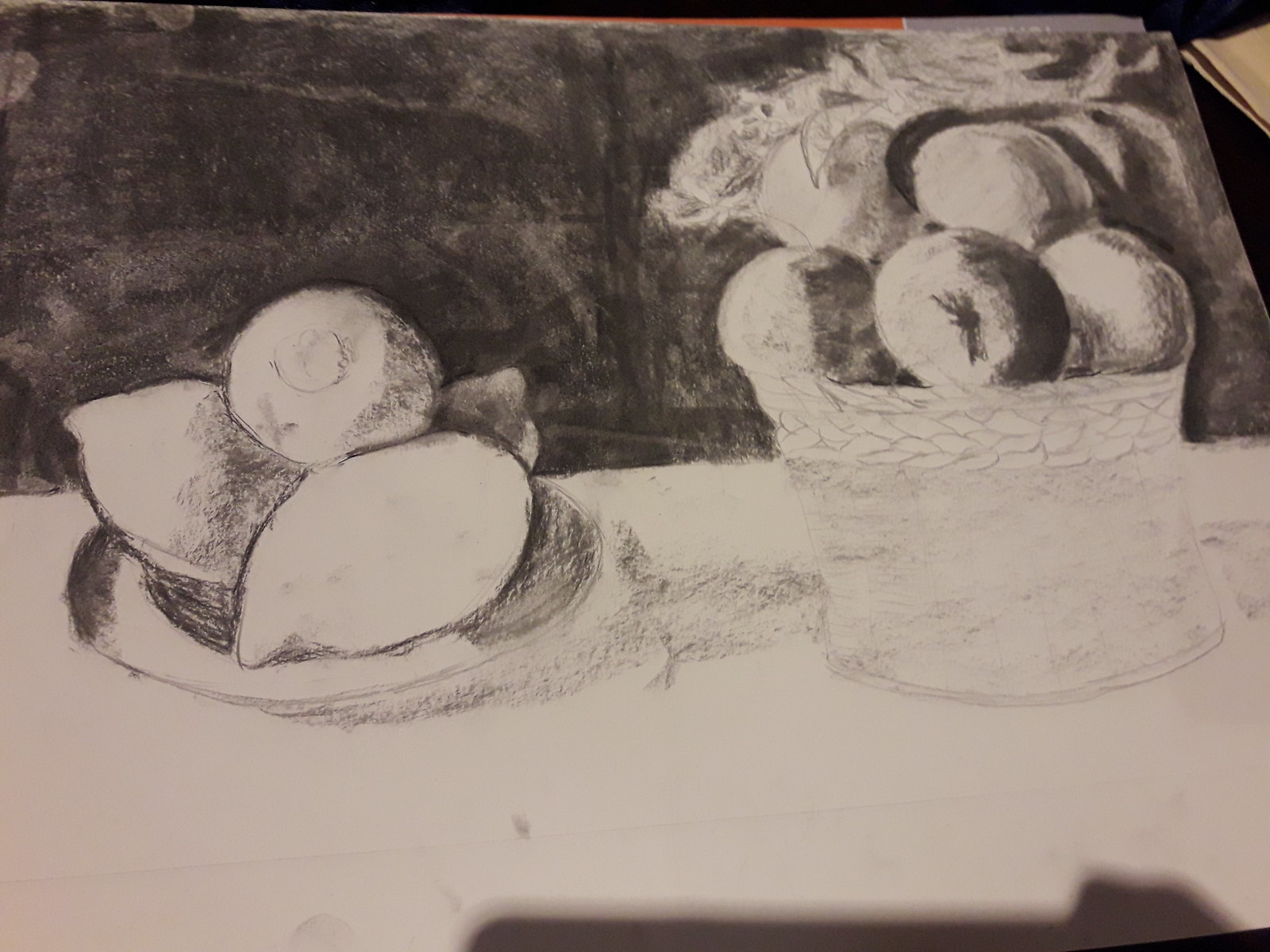This image is a detailed black and white charcoal or pencil sketch. The top half features a dark gray, almost black background, likely representing a wall. In contrast, the lower half of the sketch represents an off-white table, lightly shaded with gray in various spots. On the left side of the table, there's a white plate with shading on the sides, making it appear three-dimensional. The plate holds four lemons, intricately arranged with detailed shading: one points left, one angled slightly down and to the right, another faces the viewer, and the fourth points up to the right.

To the right of the plate is a wicker-like basket or pot that stands upright, filled with rounded fruits, possibly apples or tomatoes. The basket shows detailed texturing and has a few fruits sitting in its base. The foremost fruit in the basket is round with a stem pointing towards the viewer, resembling a tomato. Above it, there are two more rounded fruits, each accented with shading and what seem to be leaves on top. Beneath the sketch, captured in the image, is the shadowed silhouette of a hand holding an iPhone, indicating that this is a photograph of the drawing.